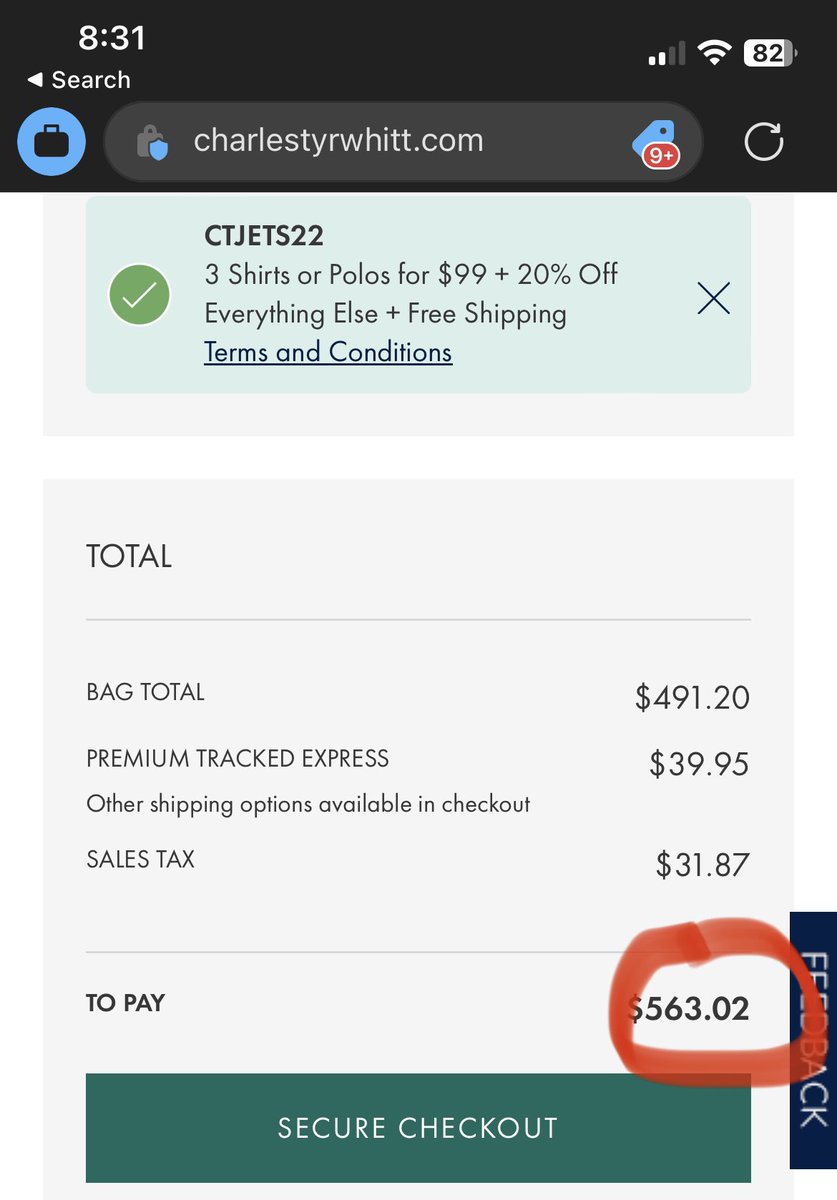The image displays a screenshot of a webpage from charlestyrwitt.com. At the top, from left to right, the time is shown as 8:31. Adjacent to it is the text "search" alongside an icon resembling a black briefcase. In the search bar, the URL "charlestyrwitt.com" is visible. To the far right, the battery life of the device is displayed at 82%.

Beneath this black navigation bar, there is a light blue promotional banner stating "CTJETS22. Free shirts or polos for $99 plus 20% off everything else plus free shipping." The terms and conditions are highlighted in blue text.

Below the promotional banner is a light gray box containing the breakdown of a shopping cart total. The details are as follows:
- **Total:** 
  - **Bag total:** $491.20
  - **Premium tracked express shipping:** $39.95
  - (Other shipping options available at checkout)
  - **Sales tax:** $31.87
  - **Total to pay:** $563.02 (circled in red)

Finally, at the bottom of the box, there is a green banner with the phrase "secure checkout" written in white lettering.